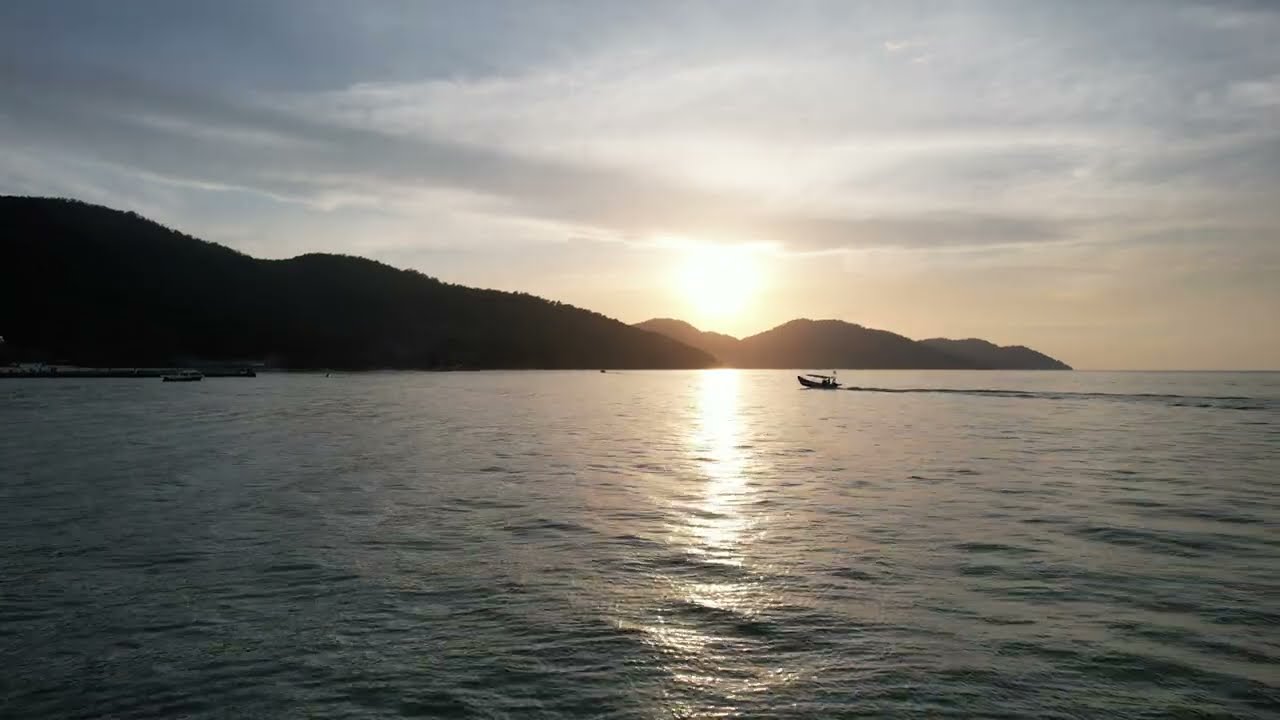The photograph showcases a tranquil scene of a large body of water, which could be an ocean, lake, or river, under a partly cloudy sky during either sunrise or sunset. The sun is positioned centrally behind a range of dark, silhouetted mountains, casting a striking reflection across the bluish-green water. The mountainous terrain spans the middle of the image, with the tallest peaks on the left. In front of these mountains, a boat with a rooftop sails towards the horizon, creating ripples in its wake. Additionally, on the left side of the image, another boat is docked by a long jetty, adding to the serene ambiance of the picture.